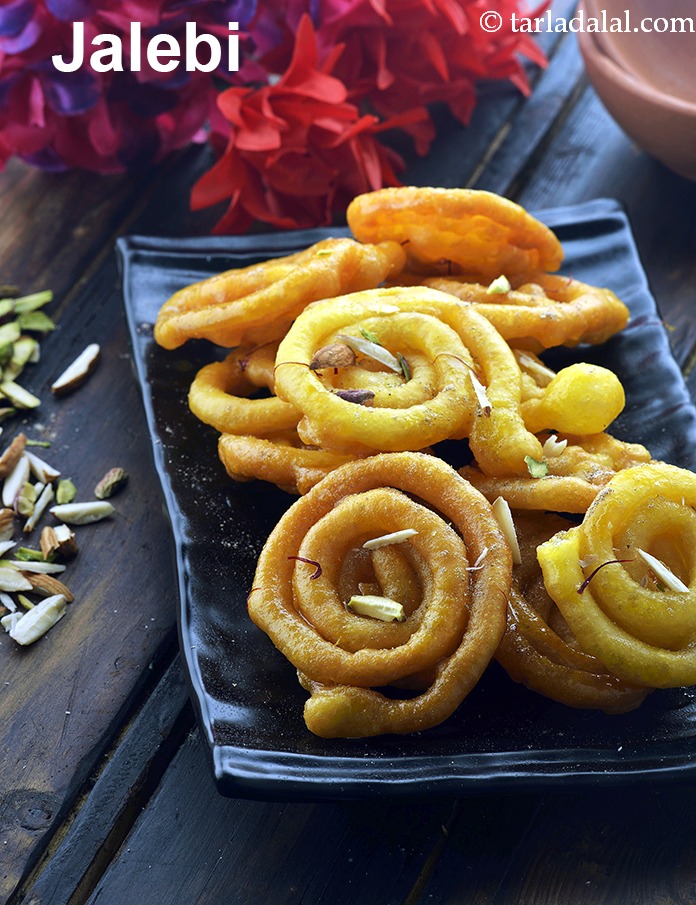In the image, a magazine cover or poster is vividly detailed against a dark wooden table that runs diagonally from the lower left to the upper right corner. At the top, the title "Jalebi" is prominently displayed in bold white letters against a dark red background in the upper left corner. Intricately detailed, the upper right corner contains a copyright notice, "TarlaDalal.com" with a copyright symbol, suggesting the image's source. The dark wood of the table juxtaposes vibrant red and purple silk-like flowers in the upper left background.

A striking black, grooved rectangular plate occupies the right middle of the image, extending from the middle toward the lower portion. On this plate, there are about 10 intricately spiraled, golden-brown jalebis that closely resemble onion rings, arranged in an overlapping pattern. The dessert is garnished with what appear to be shaved almonds, which are also scattered on the table to the left side of the plate, adding a mix of beige, green, and brown hues. The jalebis exhibit a finely detailed texture, with circular borders and tightly wound centers. The table's weathered dark brown or black wood has visible splits, accentuating an antique feel.

In addition to this, the lower right corner of the plate showcases lighter golden-colored fried foods akin to onion rings, while darker, long spiral pieces with ball-like ends of a slightly deeper brown gold hue are situated alongside. Above these, a similarly twisted piece with a lighter yellow tint contrasts against the dark and blue tones of the background. A light brown bowl's portion is seen at the top right corner, blending into the rich array of textures and colors in this vibrant culinary presentation.